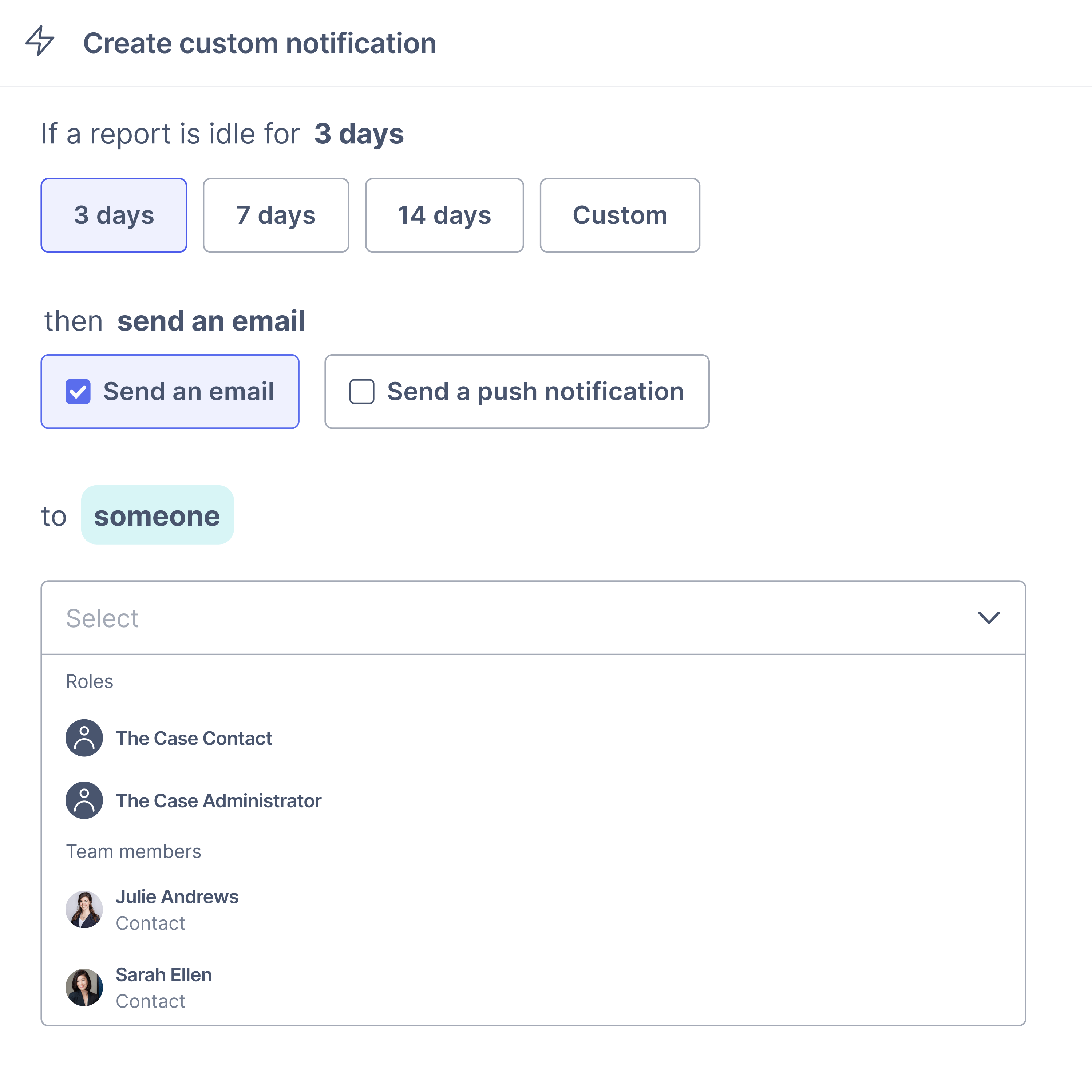**Detailed Caption:**

The screenshot features a white background. In the upper left-hand corner, there is an image of a gray-outlined hourglass, tilted slightly to the left. To the right of this image, the text "Create Custom Notification" is displayed in black font. 

A faint, horizontal light blue line separates this header from the main content below. The next section starts with black text: "If a report is idle for three days," with "three days" emphasized in bold. Directly beneath this text are four rectangular buttons arranged horizontally. The first button, labeled "Three Days," is in bold with a blue background, indicating it is selected. The subsequent buttons are labeled "Seven Days," "14 Days," and "Custom," in gray text.

About three lines further down, bold black text reads "Send an Email." Below this instruction are two rectangular options. The left button displays "Send an Email" in black text with a blue square containing a white checkmark to its left, indicating it is checked. The adjacent button reads "Send a Push Notification" in black text but is not checked; its associated checkbox is empty.

Approximately four lines down, gray text reads "To" followed by the bolded black text "Someone," which is placed on a blue rectangle highlighting it. Next, a larger rectangular field outlined in gray appears, with the word "Select" at the top and a drop-down arrow on the right side.

A gray horizontal line separates the "Select" area from the "Roles" section beneath. Under "Roles," there are two profile icons: one labeled "Case Contact" and the other "Case Administrator."

Further down, under the "Team Members" category in gray text, two profile icons represent team members: "Julie Andrews" and "Sarah Ellen."